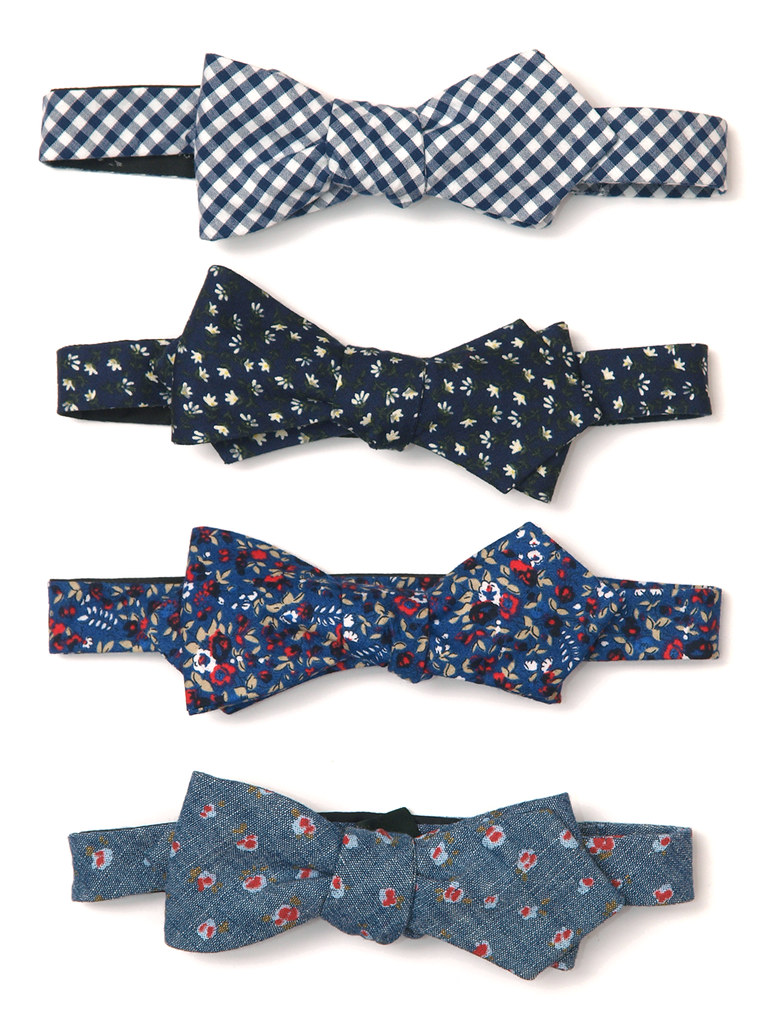In this image, we see four bow ties visually organized in a vertical stack against a plain white background. The topmost bow tie features a black and white checkered design with a diamond pattern angled at 45 degrees. Below it, the second bow tie is black, adorned with small white leaf or flower-like designs. The third bow tie is navy blue with a multicolored pattern comprising red, white, and black markings, possibly depicting flowers. At the bottom, the fourth bow tie is a light denim blue, decorated with small red and white floral shapes. All four bow ties are the type that wraps around the neck rather than being clip-ons.